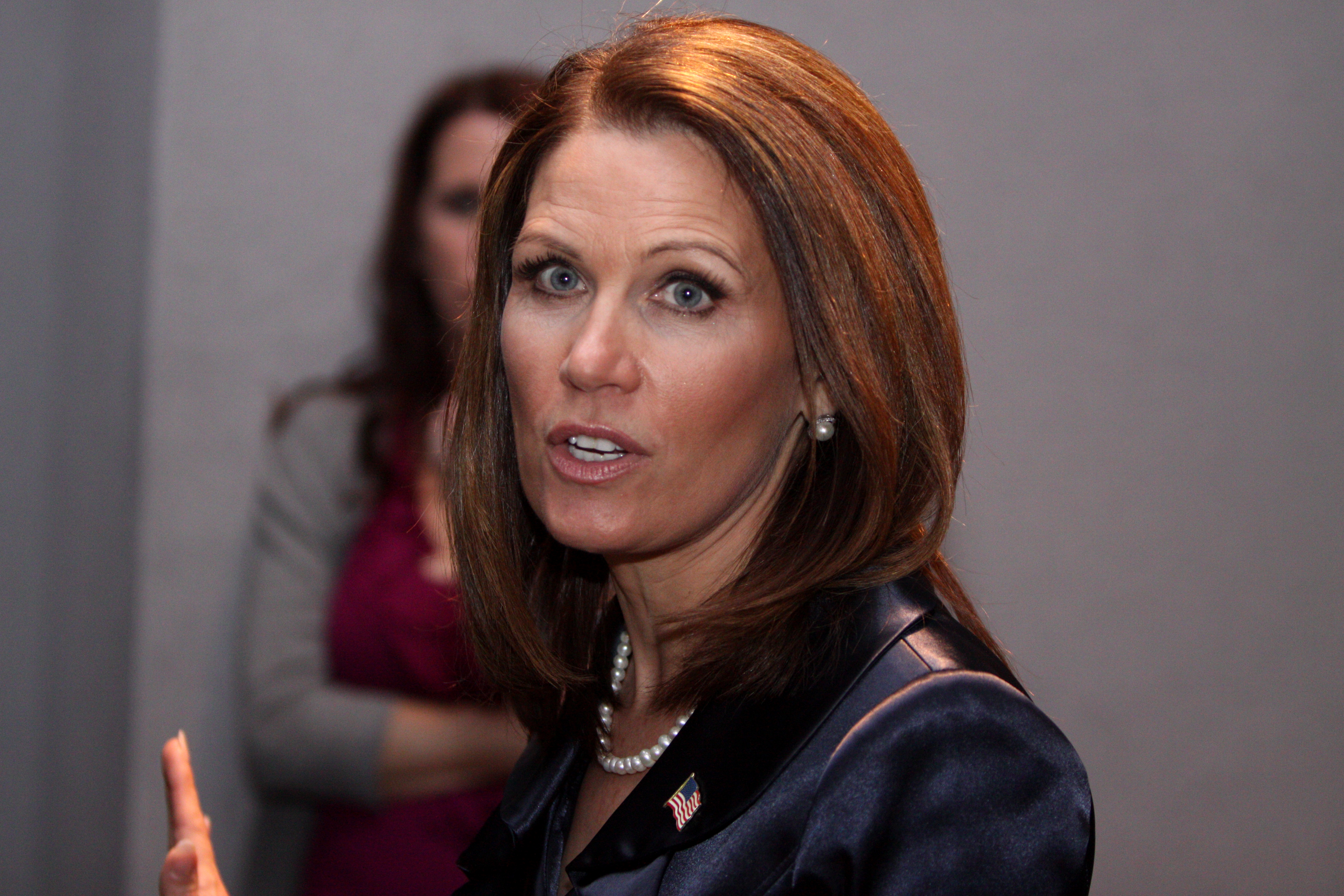This close-up portrait captures a fair-skinned Caucasian woman with auburn red hair, appearing to be in her late 20s. She stands at a three-quarter angle facing left, but her head is turned to the right, gazing directly into the camera. Her thick, straight hair is parted on the right and cascades just below her shoulders. She wears professional makeup with highly arched reddish auburn eyebrows and blue eyes accentuated by thick black eyelashes. Her mouth is slightly open as if she's speaking.

Dressed in a black V-neck jacket, she accessorizes with a white pearl necklace adorning her exposed throat and upper chest, as well as small stud earrings. A prominent detail is the American flag pin on the left lapel of her jacket. Although mostly cut off by the lower part of the image, her left hand is slightly raised, with the tops of her fingers visible at the bottom left corner.

In the blurred background stands another Caucasian woman with long, dark hair, dressed in a red shirt open at the neck and covered by a gray-sleeved garment. Her face is indistinct, and she has her arms folded over her midriff. The background itself is a blank white wall, which does not feature any distinguishing marks or letters.